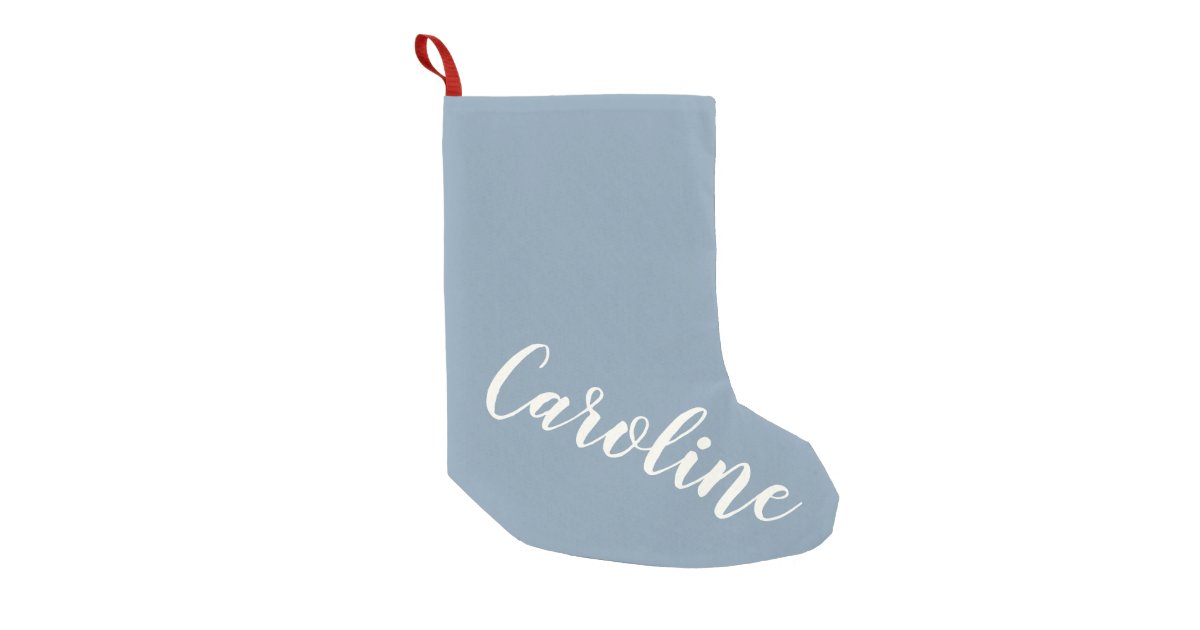This image features a light bluish-gray Christmas stocking set against a plain white background. The stocking, with a slight baby blue tint, is oriented to the right and detailed with smooth curves and angles suggesting it's sewn from a soft material. At the top left, there's a red ribbon loop for hanging. In elegant white cursive text, the name "Caroline" is inscribed in a continuous line starting from above the heel and extending towards the toe. The overall design hints at a personalized, possibly machine-embroidered or painted stocking, adding a touch of festive charm.